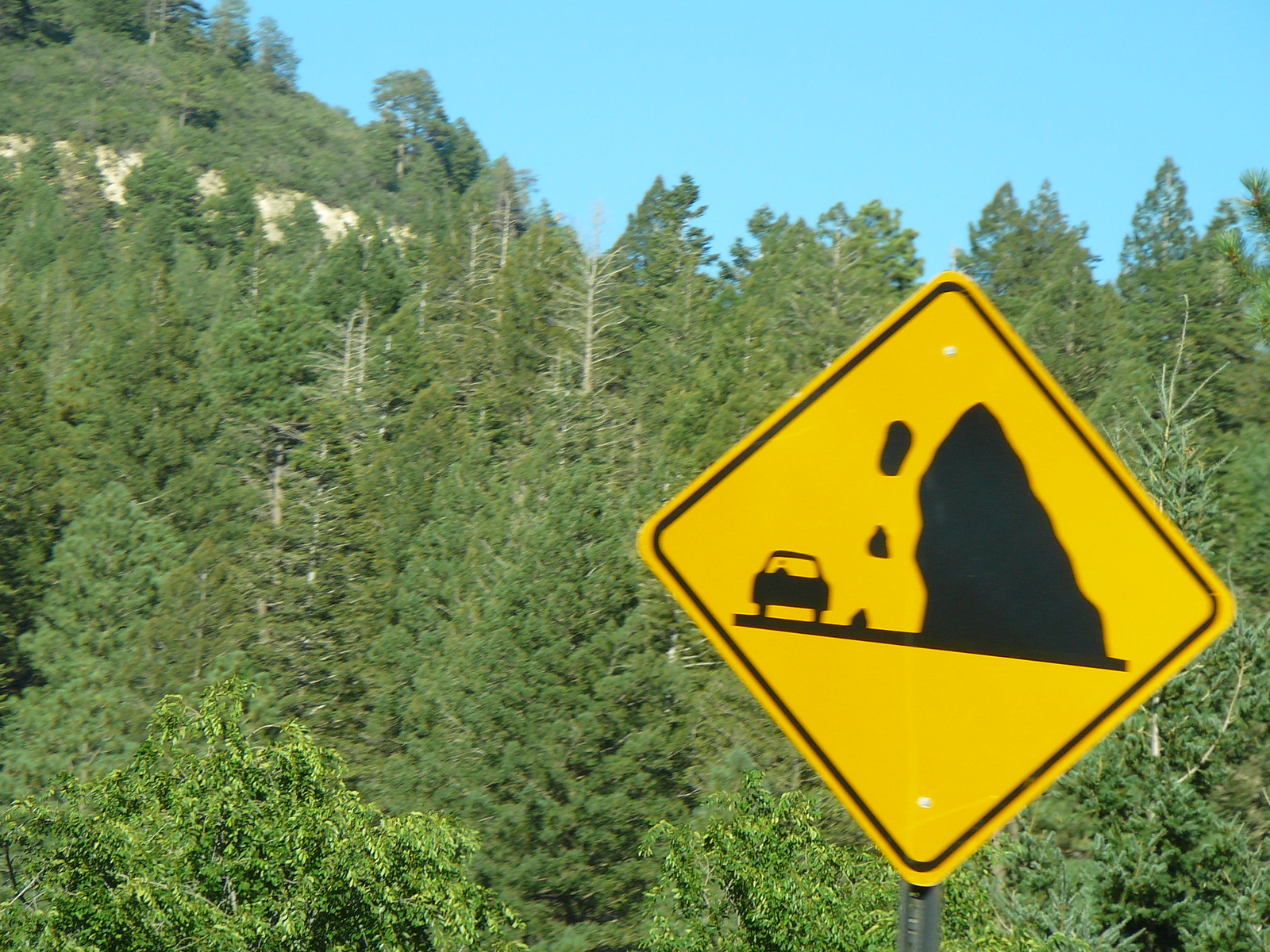The photograph showcases a roadside scene adorned with a prominent warning sign. The sign, positioned centrally, is vivid yellow and features an image of a mountain with three rocks tumbling down, alongside a depiction of a car, indicating the possibility of falling rocks in the area. This cautionary marker is affixed to a sturdy silver metal post. The background is a lush, dense forest with numerous trees, creating a woodland ambiance. To the left of the frame, a small mountainous hill subtly rises, adding depth and natural beauty to the landscape.